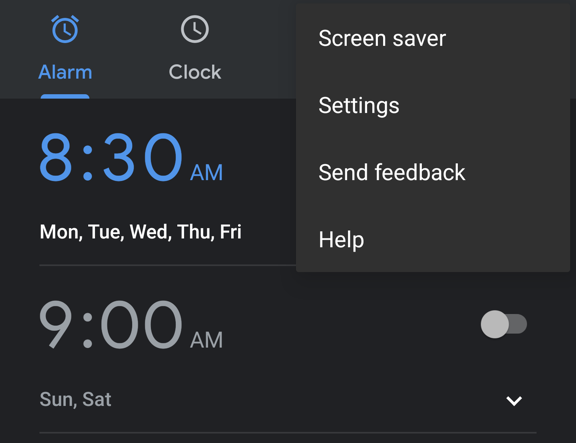The image depicts a mobile device screen, likely from a smartphone. The background is predominantly black with some dark slate gray elements. In the top left corner, there is a blue "Alarm" label underlined with a blue line, and next to it, a white "Clock" label.

On the right side, a pull-down menu is visible, displaying options: "Screensaver settings," "Send feedback," and "Help."

The central section features two alarms. One alarm, set for 8:30 a.m., is highlighted in blue and specifies the days "Monday, Tuesday, Wednesday, Thursday, Friday" underneath in white text. Beneath this, a second alarm set for 9:00 a.m. is shown in white, applicable to "Saturday, Sunday," with a gray and white toggle switch on the right side indicating it is turned off. 

Below the second alarm, there is a dropdown menu, presumably for selecting specific days of the week. The colors used throughout the interface include shades of blue, white, gray, black, and a near-black slate gray. Overall, the screen appears to be a part of an alarm setting interface designed for configuring weekday and weekend alarms on a mobile device.